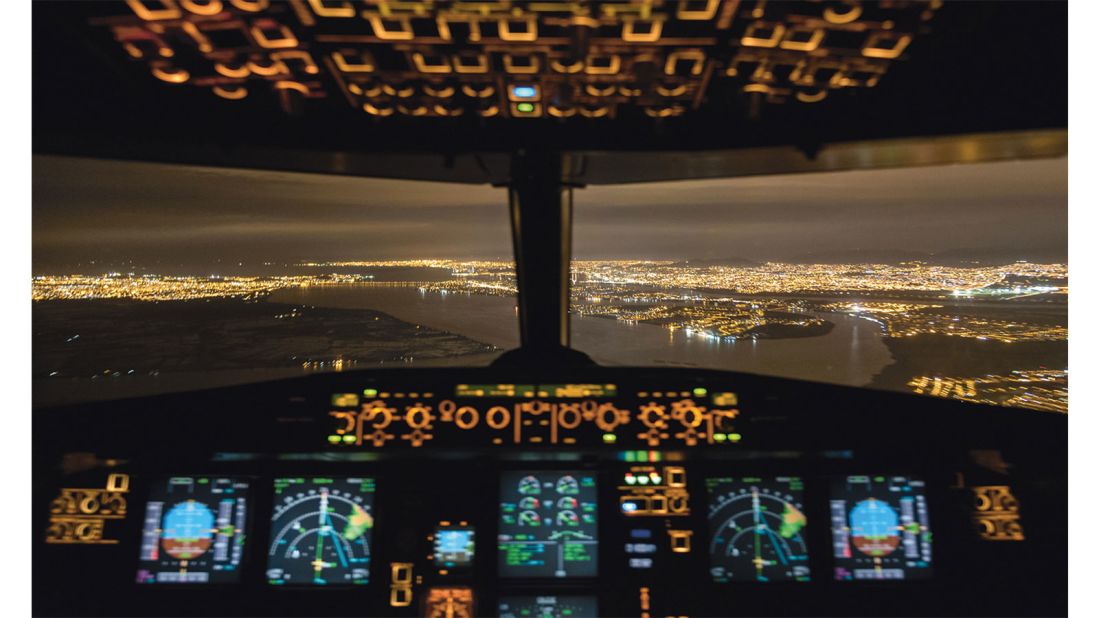In the image, we see the cockpit of an aircraft at night, captured from the pilot's point of view. The focal point is the sprawling cityscape illuminated by countless lights, stretching from the left to the right of the image and interspersed with dark patches indicating bodies of water. The sky above is pitch black, providing a stark contrast to the vibrant city lights below. The cockpit itself appears blurry, but it is filled with an array of dials, speedometers, gauges, and buttons—some of which glow orange. The upper part of the cockpit features numerous switches and lights. The windshield is segmented, offering a panoramic view of the cityscape and waterways that lie ahead. Despite the blur, the intricate layout of the cockpit's controls is discernible, adding depth to the photograph and highlighting the complexity of the aircraft.